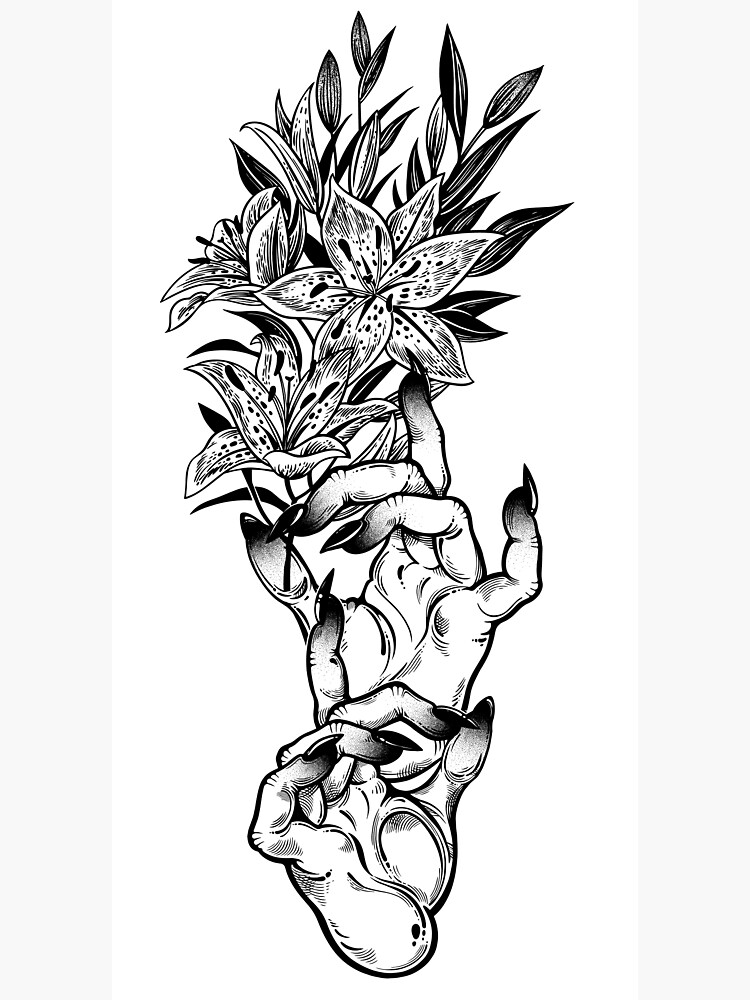This image is a black and white line drawing that appears to be a design for a tattoo or sticker. It is presented in a vertical, portrait orientation. The focal point features two gnarled, witch-like hands adorned with long, sharp fingernails painted a dark color. The hands are positioned one above the other, both with palms facing the viewer. The bottom hand has its pointer finger straight while the other fingers are bent; the top hand has its thumb and pinky finger straight, with the remaining fingers bent. Above these intriguing hands are three prominently open lilies, arranged with two on the left and one facing forward on the right. Behind and above these lilies are additional unopened lily buds and leaves, creating a layered, botanical aesthetic. The entire composition is set against a stark white background, emphasizing the intricate black and white line work, making it reminiscent of traditional tattoo art.